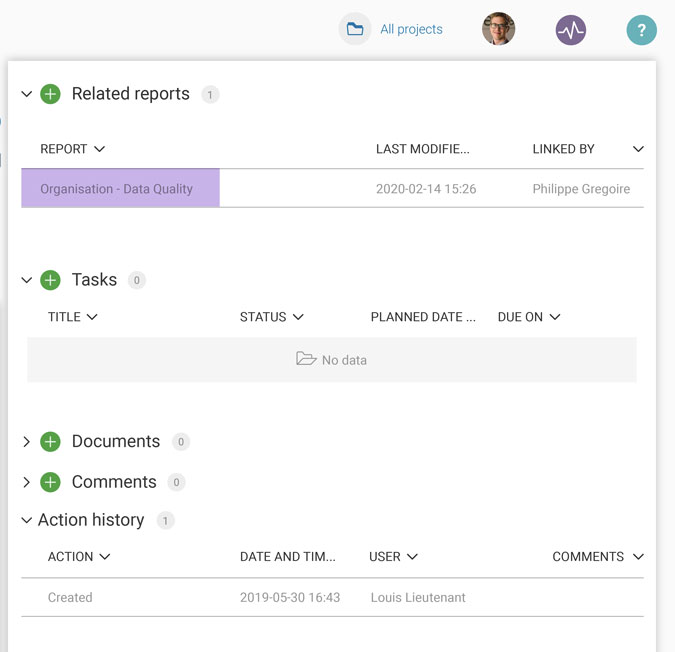The image features a user interface with a neutral gray background. At the top, a white square houses the heading "All Projects" accompanied by a circular icon with a file folder. Below, the interface displays a profile picture next to a purple circle that contains a white chart and line graph icon. A teal circle with a white triangle follows, indicating another section or button.

Additionally, the layout includes a segment labeled "Related Reports," featuring a green circle with a white plus symbol and a gray circle displaying the number one. Underneath, there are categories such as "Report," "Organization," and "Data Quality."

Highlighted in a purple rectangle is text that reads "Last Modified... 2022-14-15 15:26 by Felipe Gregorio." This purple rectangle denotes recent changes or updates to the document.

Further down, the interface lists "Tasks" with a gray circle showing zero tasks. Columns for "Title," "Status," "Plant Date," and "Due On" are present, though the section displays a gray rectangle indicating "No Data."

The image also includes sections titled "Documents" and "Comments," each paired with green circles featuring white plus symbols and both labeled zero.

At the bottom, there's an "Action History" section marked by a gray circle with the number one, alongside "Action Created Date and Time...".